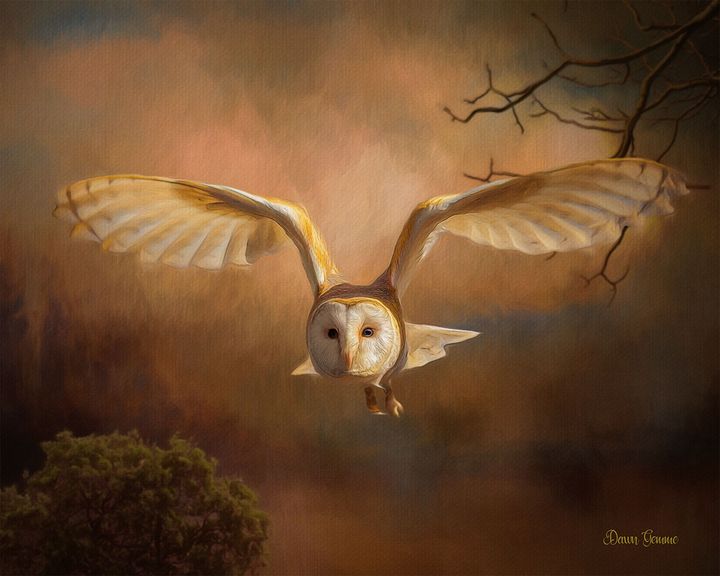The image is a detailed painting of an owl in flight, heading directly towards the viewer with its wings extended upward. The background features a blend of hazy browns, greens, reddish hues, and grays, evoking a natural sky-like setting. In the top right-hand corner, there are bare branches of a tree, while the bottom left-hand corner displays the top of a bush or tree. The owl is positioned near the mid-center of the composition, characterized by its striking white face with black eyes and a hint of yellow-gold around its beak and facial frame. Its body showcases a brownish-gold tint, and the wings, tipped with white and interspersed with golden hues, add dynamic movement to the painting. The overall scene exudes a sense of realism combined with artistic flair, resembling a serene yet captivating moment in nature. A small, unclear signature by the artist is located in the bottom right corner, possibly reading "Don Gibbrick" or something similar.